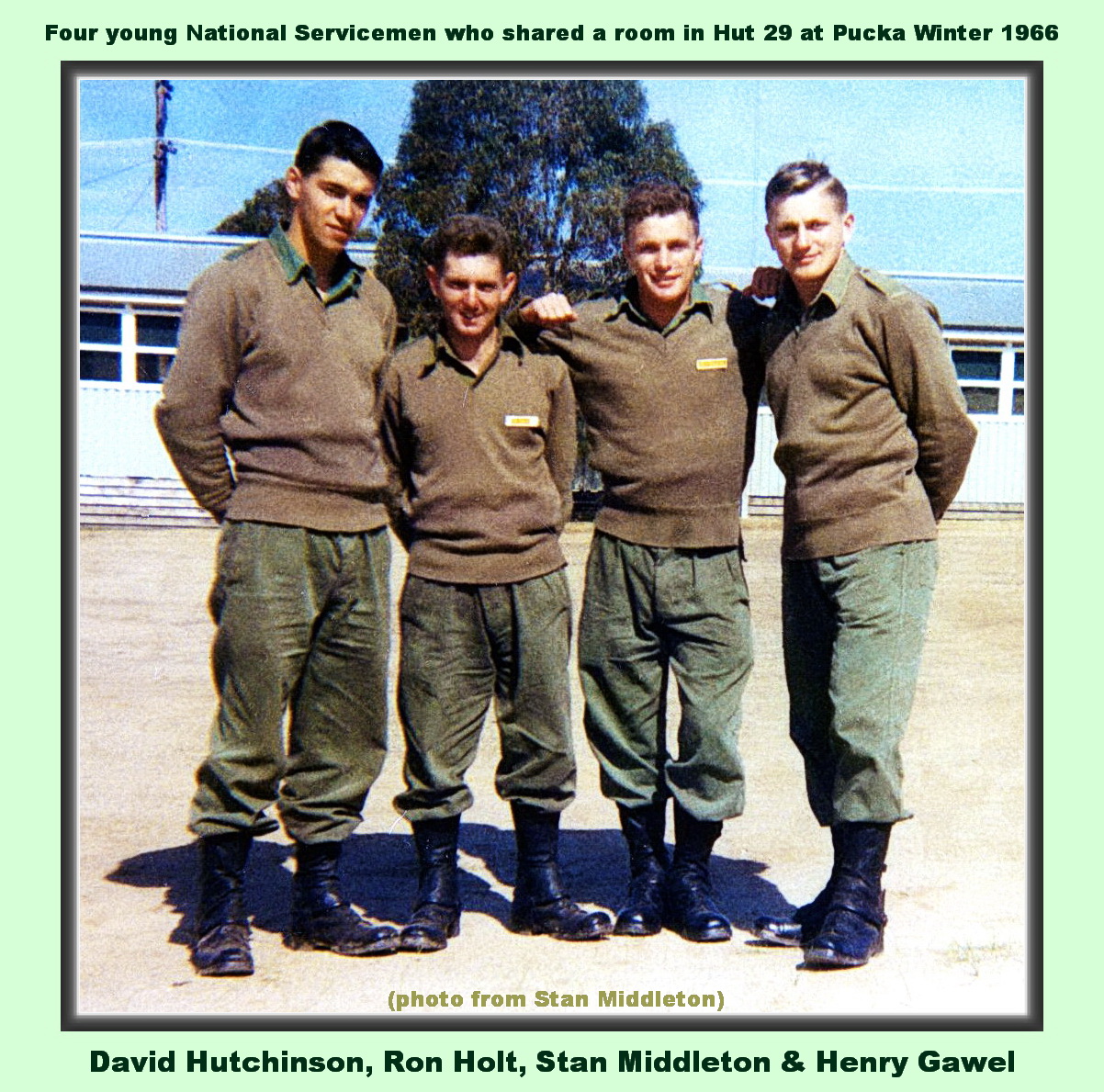This photograph, titled "Four Young National Servicemen Who Shared a Room in Hut 29 at Pucca, Winter 1966," captures four men posed together outdoors against a backdrop that includes a tree, blue sky, and a white building. The men, identified as David Hutchinson, Ron Holt, Stan Middleton, and Henry Gowell from left to right based on the text at the bottom of the image, are all dressed in matching military attire. They wear brown sweaters with collars at the neck, tan or brown pants, and black combat boots. The two men in the middle have name tags over their hearts, while the men on the ends do not. Notably, the third man from the left (Stan Middleton, as indicated by the caption and his stance in the photo) has his arms raised, resting them on the shoulders of his neighboring servicemen. The men's hairstyles differ slightly, with the first and second men having black hair and the third and fourth sporting brown hair. The scene exudes camaraderie as these young servicemen stand in formation, their expressions and posture reflecting the shared experiences of their time together in Hut 29 during the winter of 1966. A note in green text within the photo itself attributes credit to Stan Middleton for the photograph.